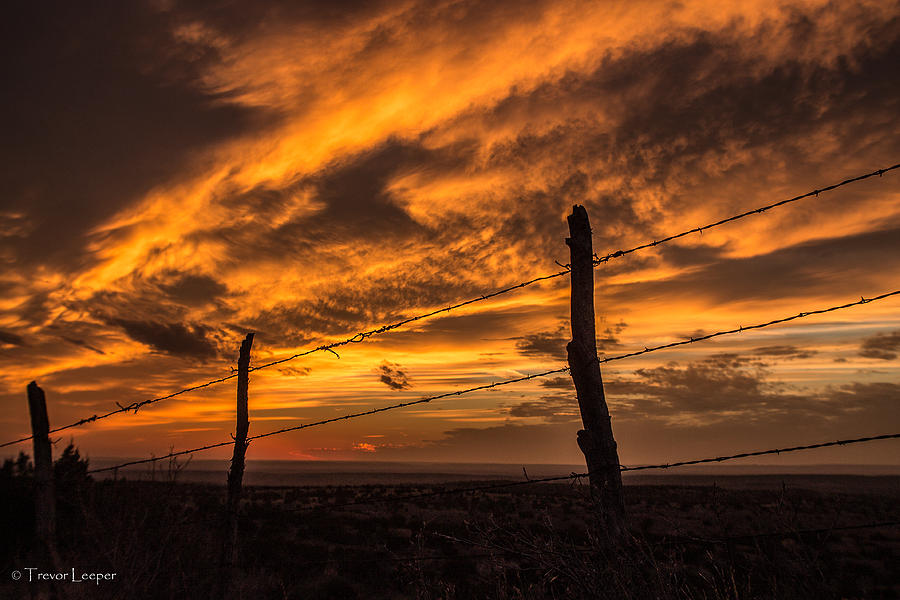A stunning photograph taken from the vantage point of someone lying on the ground captures a vivid sunset sky filled with fiery oranges, yellows, and hints of blue. The foreground features a rustic wooden fence made from rough-hewn sticks and strung with three strands of barbed wire. The ground below is a dark, prairie-like landscape with patches of dead tan grass and sandy dirt, giving an almost silhouette effect against the vibrant sky. The clouds, sparse yet dramatic, vary from bright orange and yellow hues to darker charcoal shades, intensifying the impression of a sky ablaze. The entire sky is lit with an ombre of colors, with no visible sun but an unmistakable glow indicating its presence just below the horizon. In the bottom left corner, the photograph is credited to Trevor Leeper in white font, adding a professional touch to this mesmerizing scene.